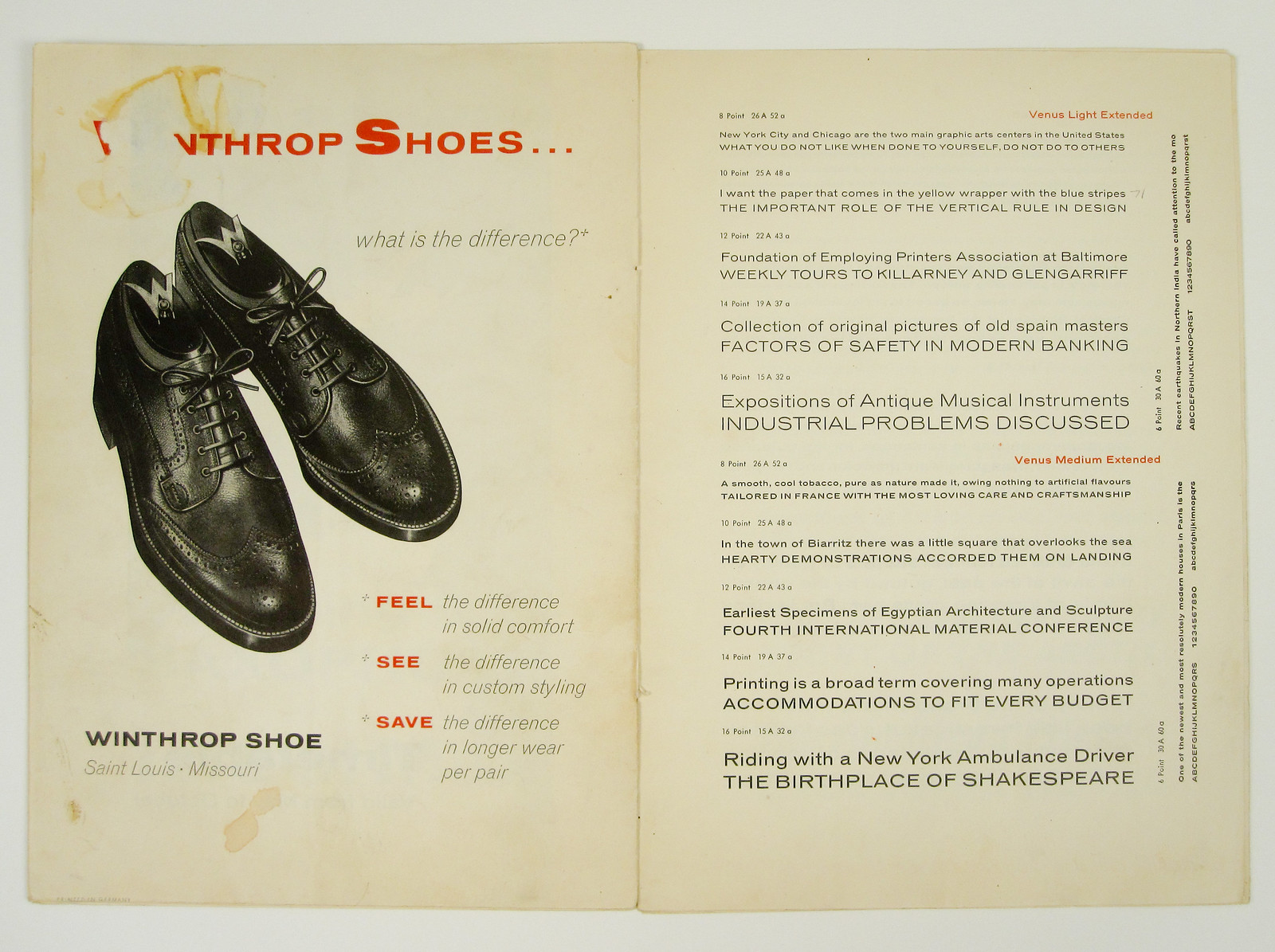The image is of an open, horizontally rectangular magazine or book spread with a white border. On the left page is an advertisement for Winthrop Shoes featuring a pair of black patent leather wingtip shoes. The title "Winthrop" appears at the top and bottom, though the letters "W" and part of the "N" at the top are washed away by a water stain. The advertisement includes the slogan in red text: "Feel the difference of solid comfort, see the difference of custom styling, save the difference in longer wear per pair." The bottom corners note locations: "St. Louis Missouri" and "New York City and Chicago are the two main graphic arts centers in the United States." On the right page, there is a dense block of text that includes varied and unrelated content, possibly excerpts or snippets from different sources, covering topics like antique musical instruments, industrial problems, and design principles. There are mentions of "expositions of antique musical instruments," and "printing in a broad term covering many operations," with additional eclectic notes about a town named Britser and references to Shakespeare's birthplace.